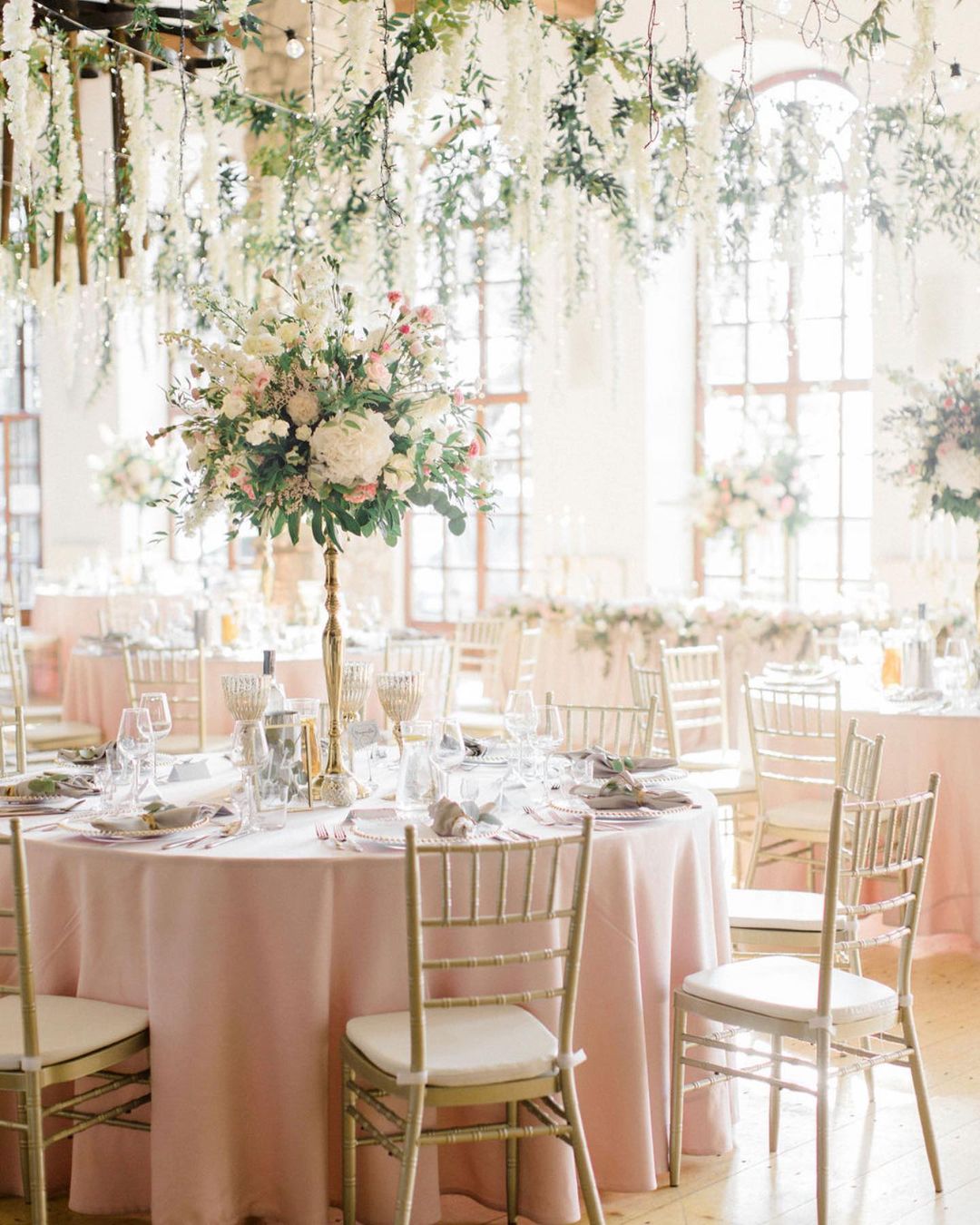This photograph captures a beautifully decorated wedding reception held in an elegant event hall. The room is filled with round tables adorned with long, pink floor-length tablecloths, creating a soft and romantic ambiance. Each table is surrounded by gold thin dining chairs with plush white or cream cushions. The centerpiece of the tables features tall, slender gold stands supporting large, round arrangements of pink, white, and green flowers, which add height and elegance to the setting.

Suspended from the ceiling are cascading designs of ivy and greenery, adding a lush, natural element to the decor. The room is bathed in natural light streaming through three large arched windows at the back, enhancing the serene and romantic atmosphere. The tables are meticulously set with wine glasses, water glasses, silverware, plates, and napkins neatly folded in rings on top of each plate.

The pale wooden or tan-tiled floor complements the overall color scheme of the room. Every detail, from the elegant crystal glassware to the thoughtfully arranged floral centerpieces, contributes to the sophisticated and inviting ambiance of the reception.